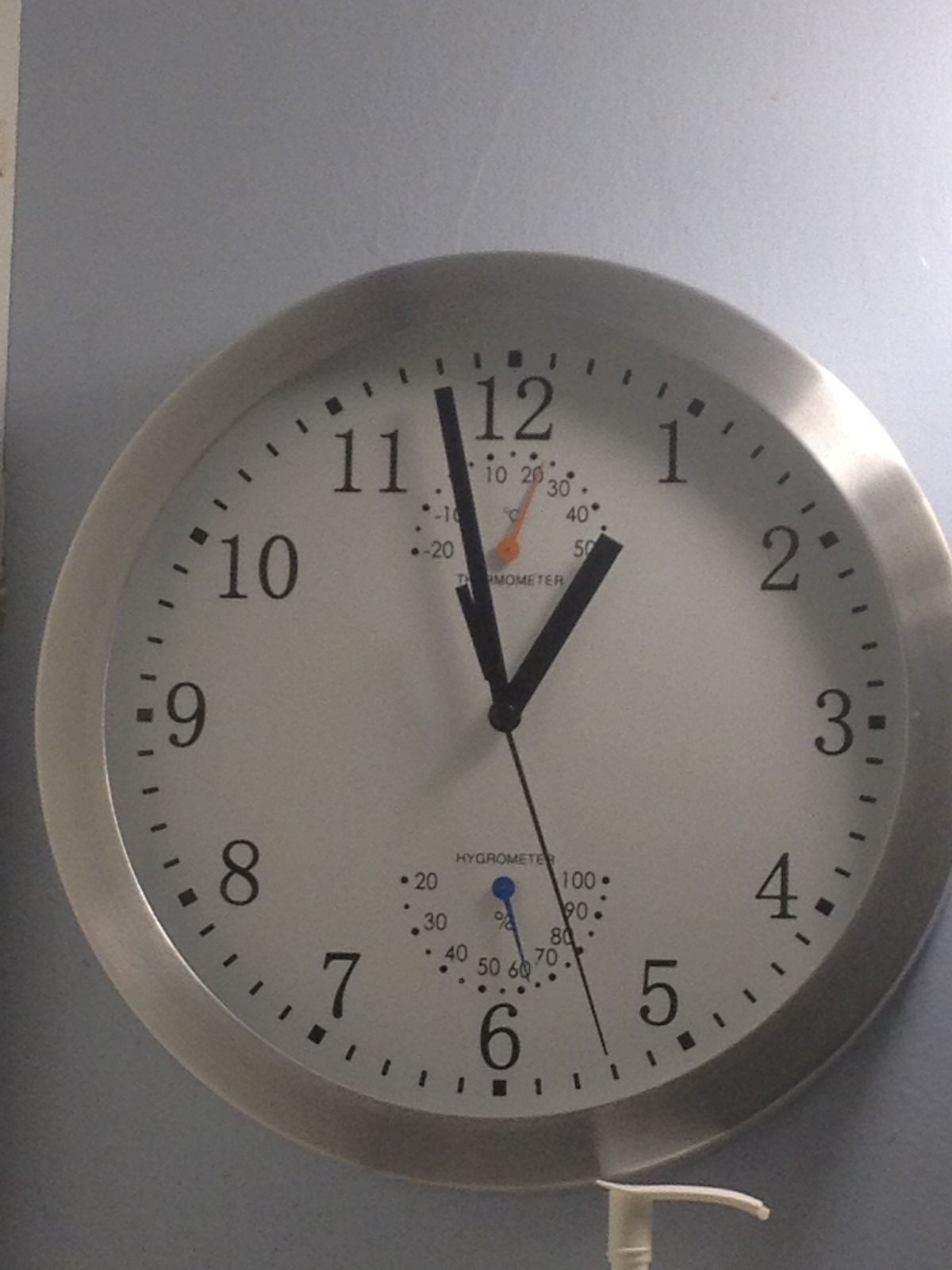This photograph captures a round wall clock mounted on a dove-gray background. The clock features a silver outer frame, which subtly reflects surrounding light. The clock face is white and prominently displays black hour and minute hands, along with large black numbers and black dash marks denoting each hour. Above the 12, there is a second set of smaller black numbers ranging from -20 to 50, accompanied by a tiny orange hand. Additionally, located above the 6, another set of black numbers from 20 to 100 is marked, which is navigated by a tiny blue hand. At the bottom of the clock, there is a white pump handle, adding an intriguing element to the overall design.